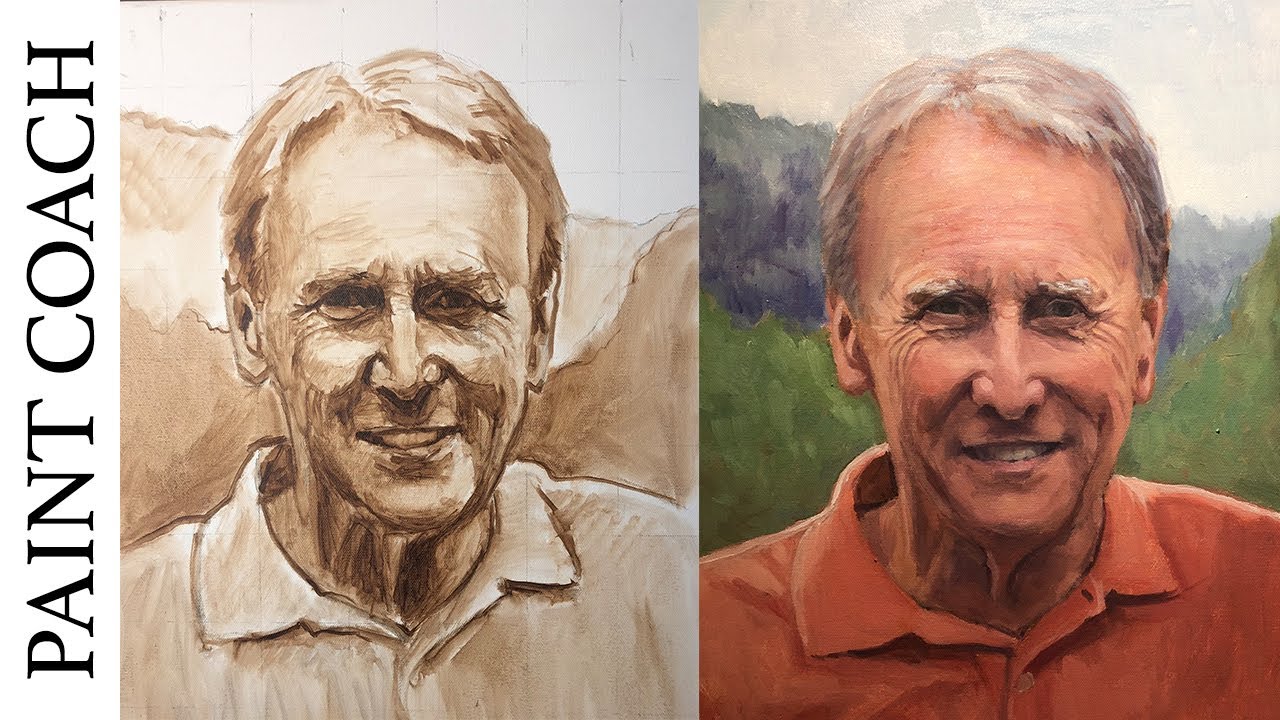This image showcases a comparison between a preliminary sketch and a finished painting of an elderly man, both displayed in picture frames. In the far left-hand corner, bold black vertical text reads "Paint Coach." The framed image on the left features a rough, monochromatic draft—either pencil or brown hues—depicting a smiling man who appears to be in his mid-sixties. He has short, silvery-gray hair, a lined face, and is wearing a collared shirt. The background is sketched with mountains and trees in a simplistic style. 

In contrast, the right frame displays the same man brought to life in a vibrant, detailed painting. He now wears a red collared shirt, and his gray hair is meticulously rendered. The background includes lush green mountains with varying shades and a light, overcast sky, giving the scene more depth and realism. The transformation from sketch to full painting highlights the addition of colors, shadows, and details that create a lifelike representation.